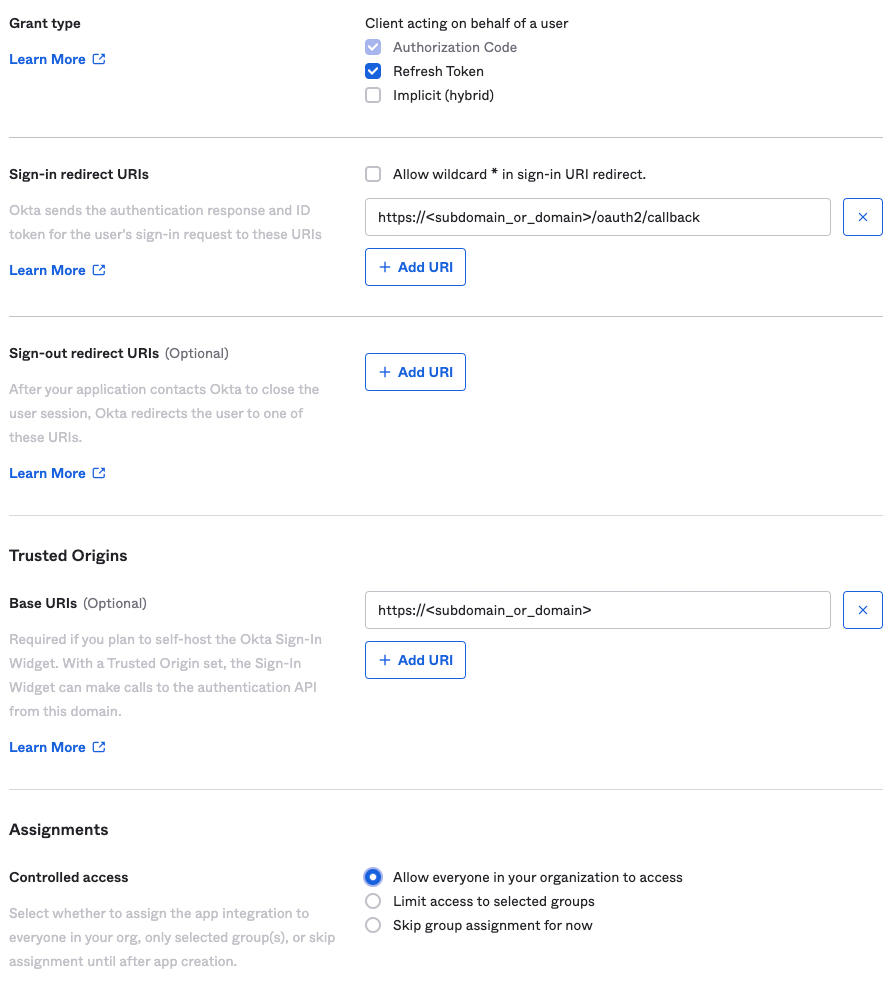In this screenshot of an information page, various settings and configurations pertaining to authorization and sign-in redirect URIs are displayed. The information is divided into sections with small font, and several terms are in black, darker blue, or grey (the grey text being too faded to read clearly).

On the left, the settings are categorized starting with **Grant Type**. Directly underneath, the options listed include:
- **Authorization Code** (ticked, pale blue)
- **Refresh Token** (ticked, dark blue)
- **Implicit Hybrid** (not ticked)

Below the grant type, the **Sign-In Redirect URIs** section explains that Okta sends authentication responses and ID tokens for user sign-in requests to specified URIs (also referred to as URLs or URIs). A learn more link is available here.

There is a checkbox for **Allow wildcard '*' in Sign-In URI redirect**, followed by a default URI: `https://subdomain.domain/oauth2/callback`. A button labeled **Add URI** allows adding additional URIs.

Next, the **Sign-Out Redirect URIs (optional)** section specifies that after Okta closes the user session, it redirects the user to one of these URIs. 

Following this is the **Trusted Origins** section, which explains that specifying base URIs is required if planning to self-host the Okta Sign-In Widget. It ensures the widget can make calls to the authentication API from the given domain.

To the right, another section labeled **Assignments: Controlled Access** appears. Here, you can configure permissions:
- **Allow everyone in your organization to access** (selected, indicated by a blue circle with a white center)
- **Limit access to select groups** (not selected)
- **Skip group assignment for now** (not selected)

No other text is provided in the screenshot. This well-organized layout ensures clear understanding and effective management of authorization and URI settings within the Okta system.